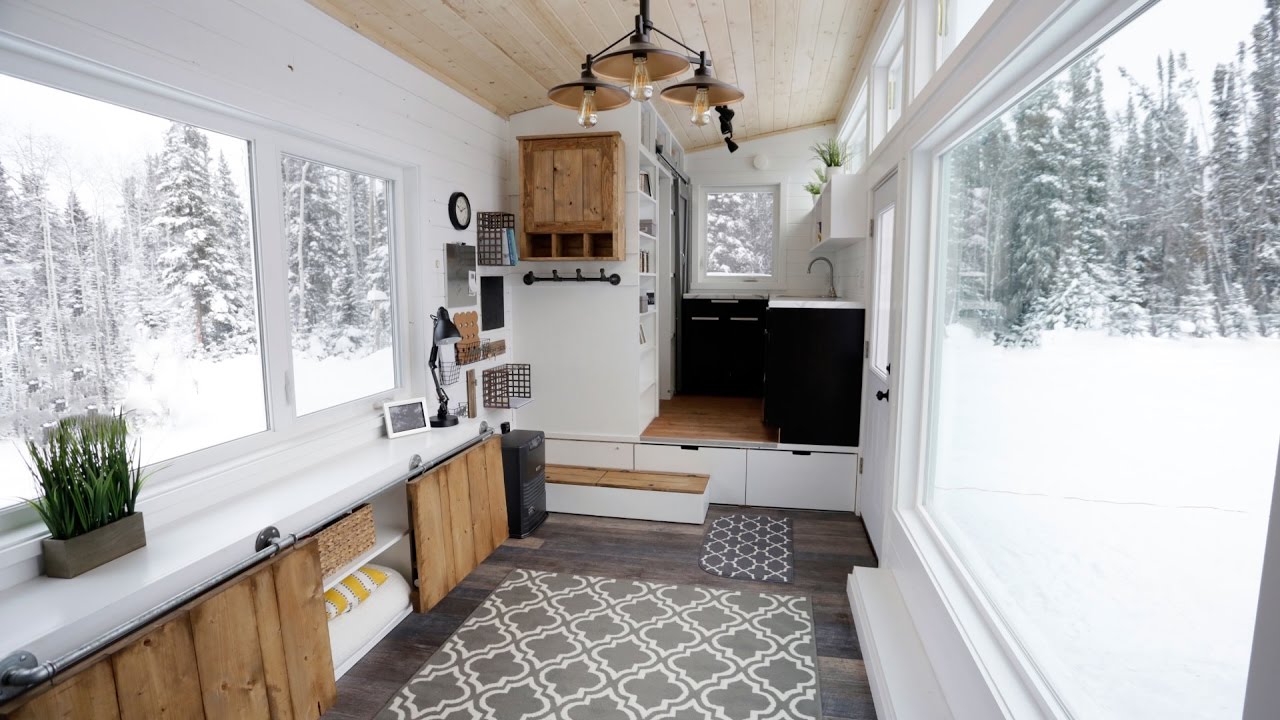This modern tiny house, possibly a custom-built RV, features large windows on either side that fill the home with natural light, accentuating its bright, open space. The white panel walls have a rustic charm, complemented by multiple light wood accents, including a blonde wood ceiling. The interior layout is streamlined and efficiently designed with storage solutions like bookshelves, drawers, and barn-style sliding doors. A cozy living room area faces a series of expansive windows, offering picturesque views of a snow-covered, pine-filled forest.

In the background, a compact yet well-equipped kitchen boasts dark countertops and powder-coated black metal accents, with a sink and possibly a dishwasher set against a barn wood-patterned floor. Above the kitchen area, angled ceilings with additional shelving house plants and other small items.

The left side of the space includes a unique wall shelf with hooks and a clock, while further along, there’s a desk area with a basket for storage. Stepping down a couple of steps leads to more drawers and a long bench that can double as additional seating or a shelf. A white door with a doorknob sits to the right, next to an oversized picture window that frames the idyllic, snowy landscape outside. The home also features a carpet on the floor, enhancing its cozy, rustic atmosphere.